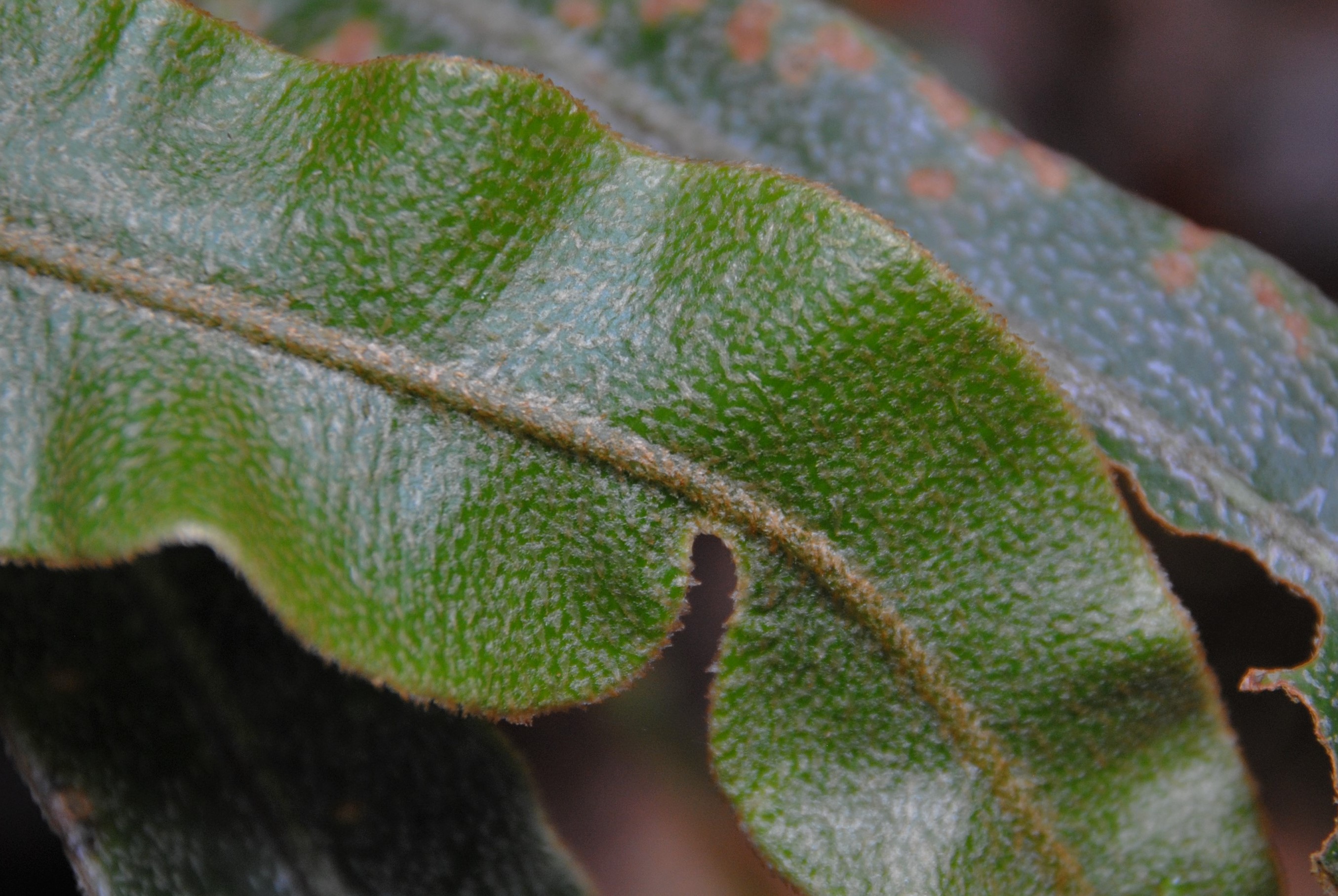This HD horizontal color photograph is a macro close-up of a wavy-edged, bright green leaf with a rough texture and brownish tones on the edges and stem. The leaf extends diagonally from the upper left to the lower right of the frame, with a central stem that is brownish in color. Small fibers resembling hairs are visible on its surface, adding to the detailed texture. In the blurred background, additional leaves from the same plant can be seen; one darker green leaf with white and brown mottling appears jagged and possibly damaged or eaten by insects. Some of these background leaves also display red specks and spots. The overall image captures the intricate details and organic shapes of the plant's leaves, with emphasis on the primary leaf's wavy and textured appearance.